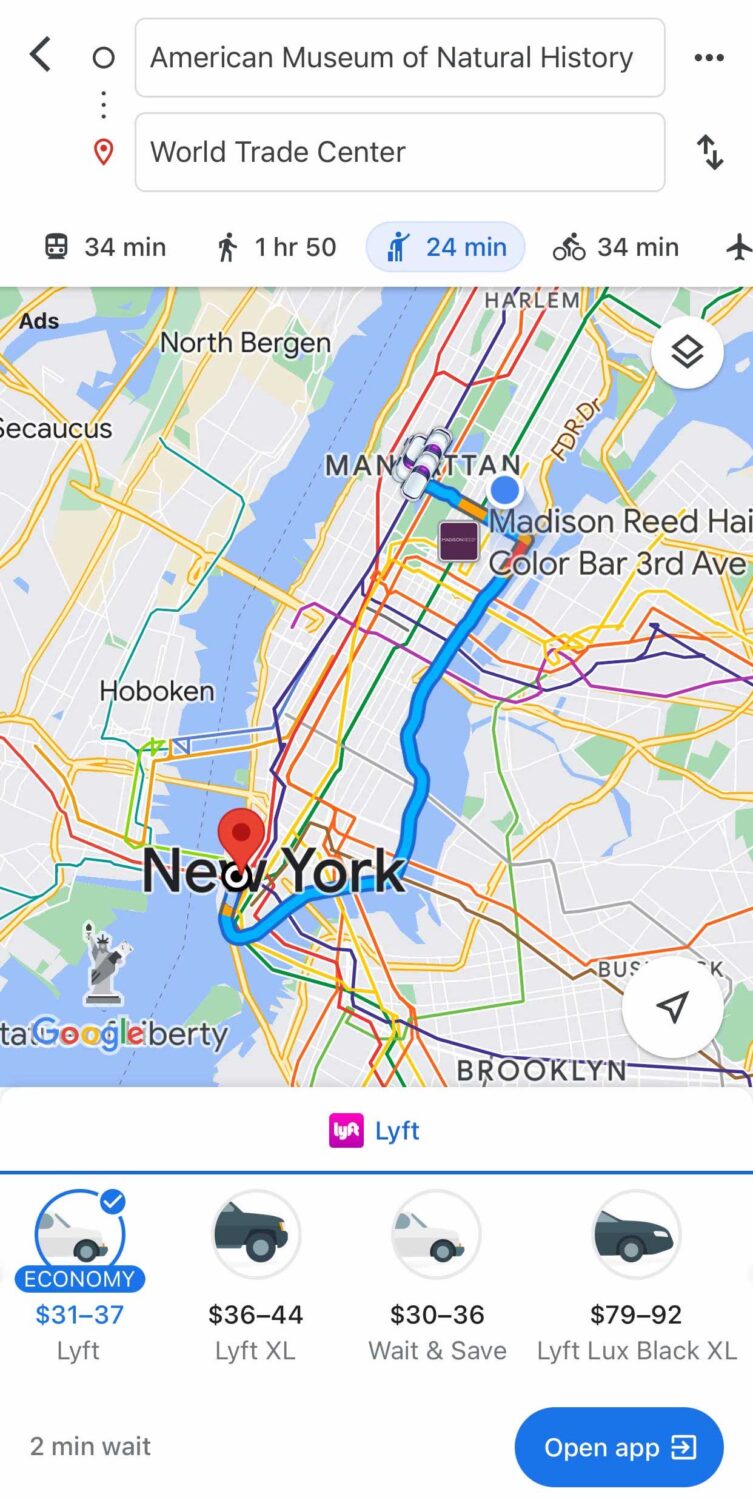This detailed map showcases lift prices and travel times between the American Museum of Natural History and the World Trade Center. At the very top, the text box reads "American Museum of Natural History," while a text box below it reads "World Trade Center." The transportation options are illustrated with icons: a bus icon indicating a 34-minute journey, a walking icon showing 1 hour and 50 minutes, and a highlighted icon of a person with a raised arm next to a suitcase indicating a 24-minute travel time. Additionally, a bicycle icon shows a 34-minute journey time.

The map below these options depicts a portion of New York City. Notable labels include "New York" in bold text near the bottom with a red pin, "Manhattan" further up, and other areas such as "Harlem," "North Bergen," "Hoboken," and "Brooklyn" in the bottom right corner. 

Beneath the map, the lift logo appears alongside four circular icons representing different vehicle types. The first icon, bordered in blue, reads "Economy" with a fare range of $31 to $37. Next is a black car icon indicating "Lift XL" with a fare range of $36 to $44. The third icon features a gray car and reads "Wait and Save" with a fare range of $30 to $36. The final icon is a black car labeled "Lift Lux Black XL" with a fare of $79 to $92 and a two-minute wait time.